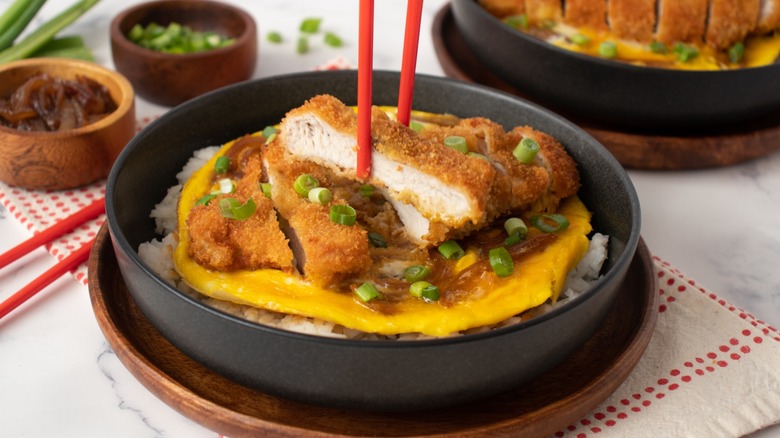Featured prominently on a white table, this image showcases a meticulously presented Asian-inspired dish centered in a black bowl atop a wooden plate. The dish begins with a bed of white rice, crowned by a circular, cooked omelette. This omelette appears smoothly beaten but not scrambled, serving as a plush base for the star ingredient: diagonally sliced, golden-brown chicken katsu. Garnished with vibrant green scallions, the chicken pieces are elegantly arranged, with one slice lifted by red chopsticks to reveal the tender, perfectly cooked interior to the camera. The bowl and plate ensemble rests on a white towel adorned with red polka dots. In the background, additional wooden bowls appear, potentially containing extra toppings like scallions, spring onions, or other garnishes, alongside another identical chicken katsu dish to the top right, all contributing to a colorful and inviting culinary scene.